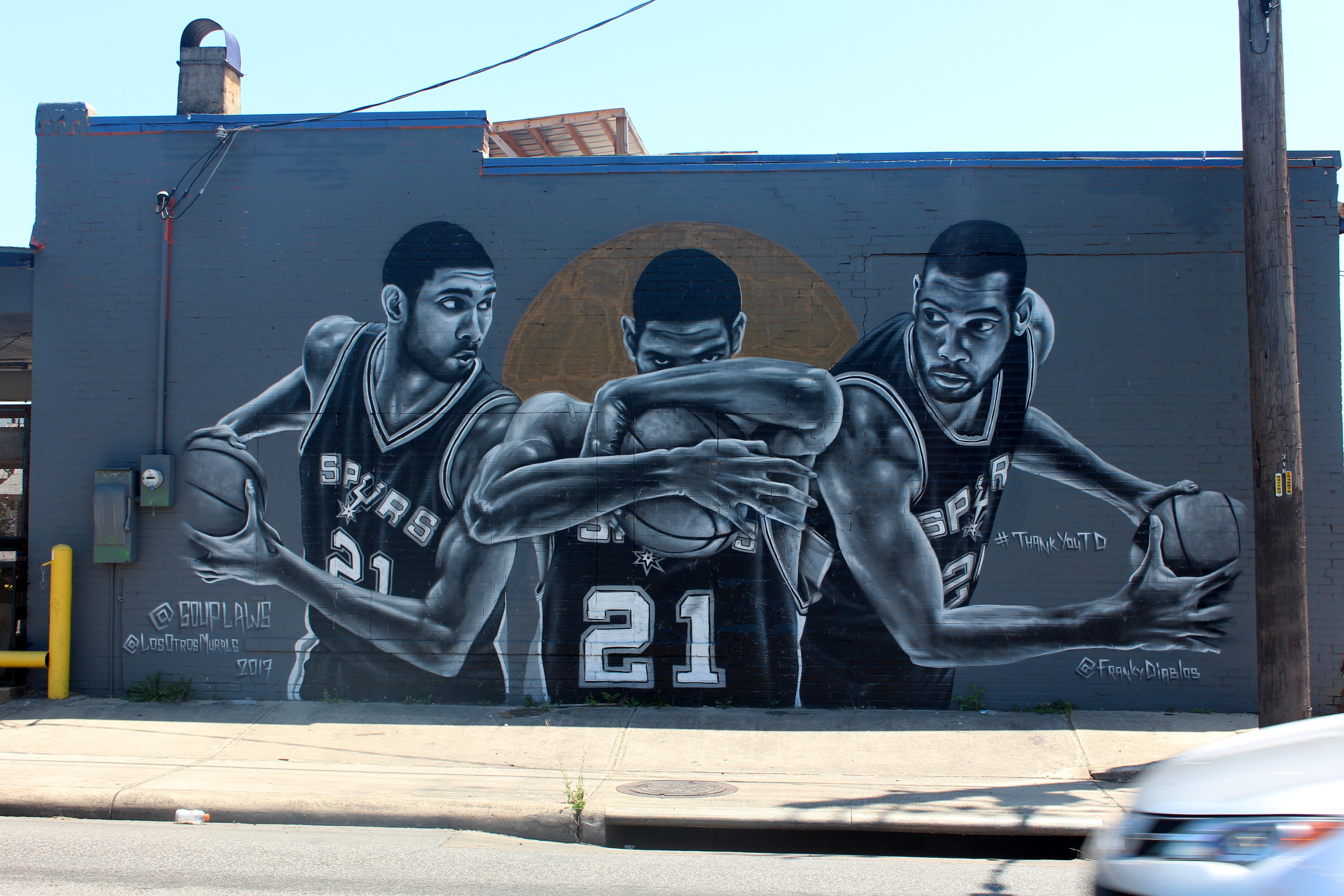This vibrant mural occupies the side of a dark blue-gray building, capturing the legendary Tim Duncan in three dynamic basketball motions. Each depiction of Duncan, donning his iconic Spurs jersey emblazoned with the number 21, shows him interacting with the ball—one where he's holding it, another where he’s tightly clutching it, and the last where he’s poised to make a move. The somber hues of blue and black dominate Duncan’s portrayals while the basketballs stand out in their bright orange contrast. Behind the central figure, a large brown circle can be seen, possibly representing a sun or moon, adding a dramatic backdrop to the composition. Additionally, notable graffiti tags read "Suplaws" and "#thankyou," marking the mural's creation as a tribute following Duncan's retirement in 2017. This detailed artwork is set against the everyday urban scenery, with a wooden utility pole, a small yellow pole, a white car edging into view from the right, and a cement sidewalk stretching out below, grounding it in the fabric of city life.